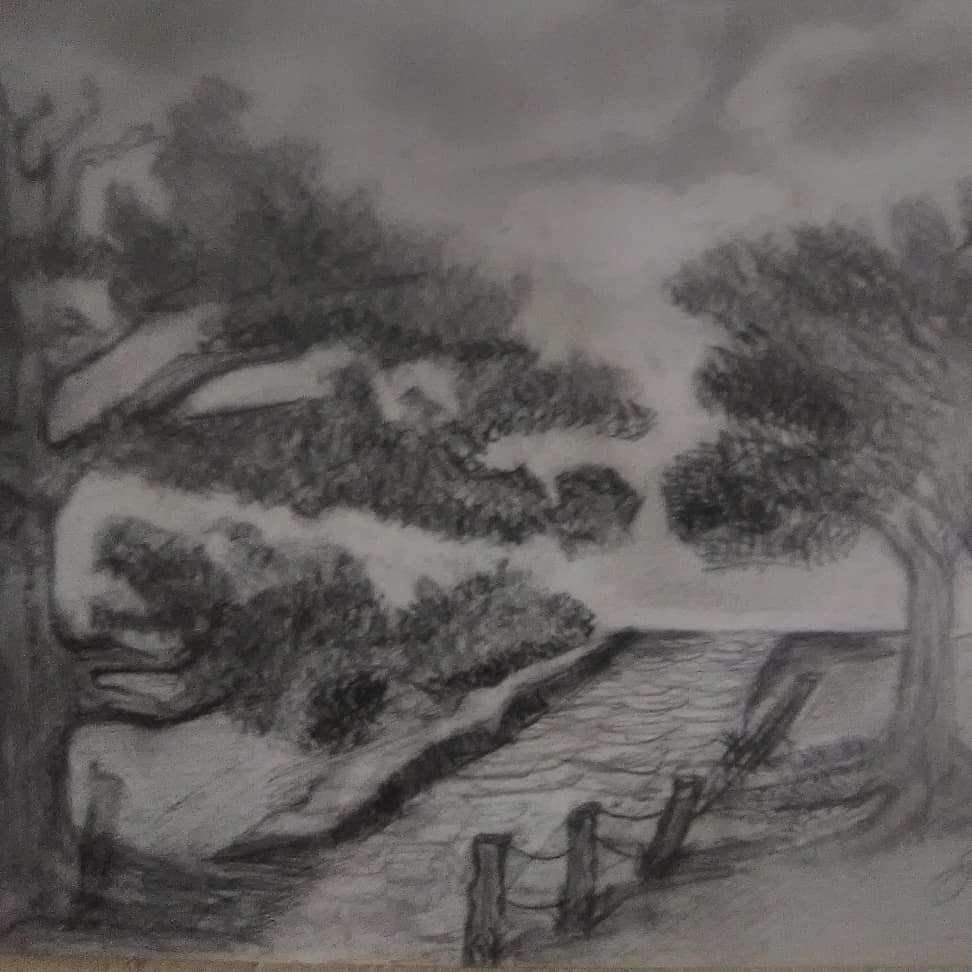This is a detailed pencil drawing rendered in shades of black, white, and gray. The focal point of the artwork is an old cobblestone road that winds its way through the scene, giving it a touch of timeless charm. On the left side of the road stands a large tree, its abundant branches and rich foliage extending gracefully over the path. To the right, another tall tree reaches skyward, adding balance to the composition. Adjacent to the cobblestone road is a dilapidated wooden fence, which further enhances the rustic atmosphere. In the background, the artist has skillfully illustrated clouds drifting across the sky, accentuating the dreamy, almost fantasy-like quality of the landscape. The overall scene evokes a sense of wonder, reminiscent of a journey down a mysterious, enchanted path.